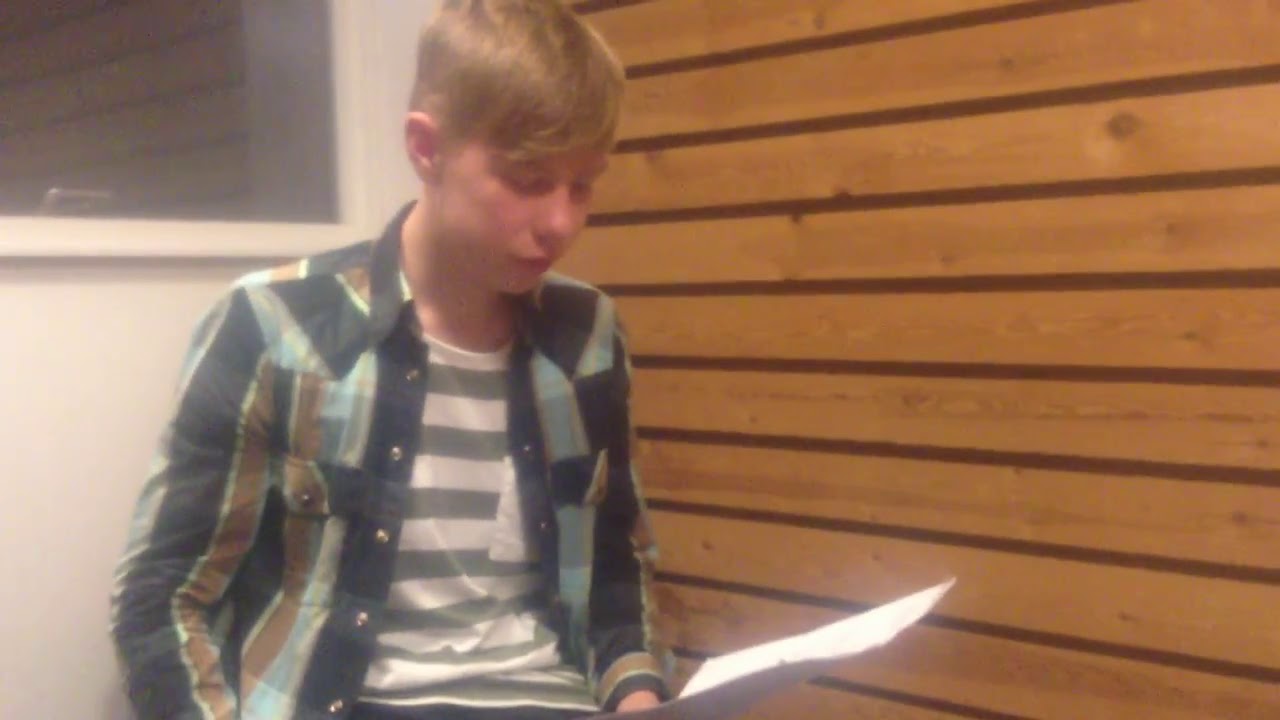In this landscape-oriented color photograph, a young teenage boy, around 10 to 15 years old, is the central focus, occupying the space from the top to the bottom of the image. The boy, who has blonde, possibly light brown hair, and a rather red complexion, is intently reading a white piece of paper held in his left hand. He is attired in a white shirt with green stripes underneath a blue and brown, possibly flannel or western-style shirt that features some orange or gold detailing. His attire gives off a casual, yet slightly rugged impression. The boy is seated inside what appears to be a house, situated in the corner of a room. Behind him to the right is a wall made of light brown horizontal wood planks, their seams darker and distinct. To the left behind him, there is a white stucco wall with a window reflecting the wood-paneled wall. The lighting in the image creates a noticeable glare on his hair and the paper, adding a slightly out-of-focus, glary quality to the photograph. The boy is fully immersed in whatever he is reading, demonstrating a complete focus that suggests the content holds significant importance to him.